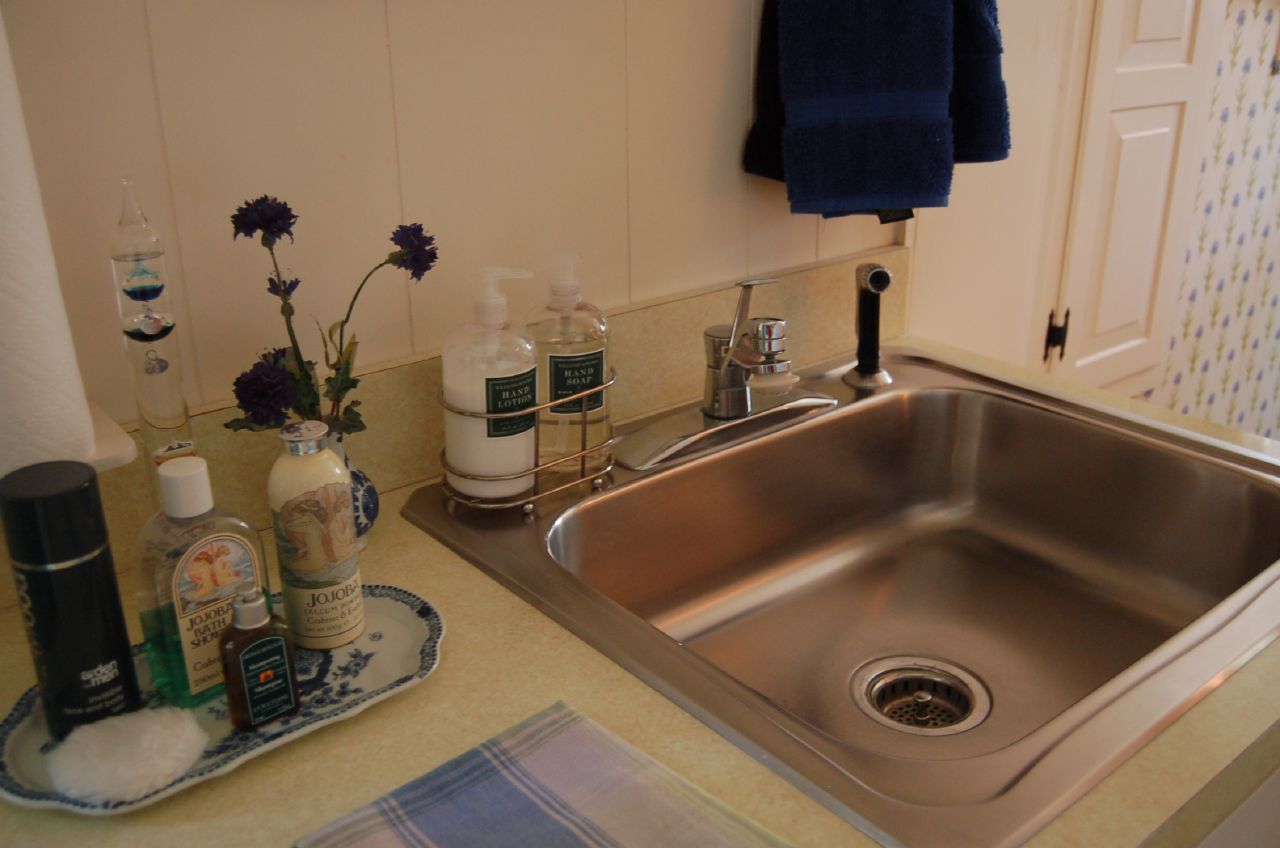The image portrays a portion of a bathroom in intricate detail. An open white door reveals a section of wallpaper adorned with a white background and blue and yellow print. Adjacent to this, a wall is painted in a very light pale pink. The countertop is a yellowish beige, extending upwards into a matching backsplash behind a long, single metal sink.

The sink itself is equipped with a black sprayer, a silver faucet, and a lift handle for water regulation. Hanging above the sink is a dark blue towel. Within the sink, the drain is visible. A small metal holder on the counter contains two large pump bottles, one with a clear liquid and another with a milky-pink substance.

Adjacent to these bottles, there's a white flower vase decorated with dark blue patterns, housing deep red flowers with green leaves. A tray that matches the vase's design holds a cotton sponge, a black can of hairspray, and three bottles of different designs and colors: a bottle with a white top, a small brown bottle with a gray top, and a beige bottle with a silver top.

In the background, a tall holder is partially visible alongside a glimpse of a shower curtain. Additionally, a smaller blue and white towel is also seen, adding to the bathroom's array of colors and textures.